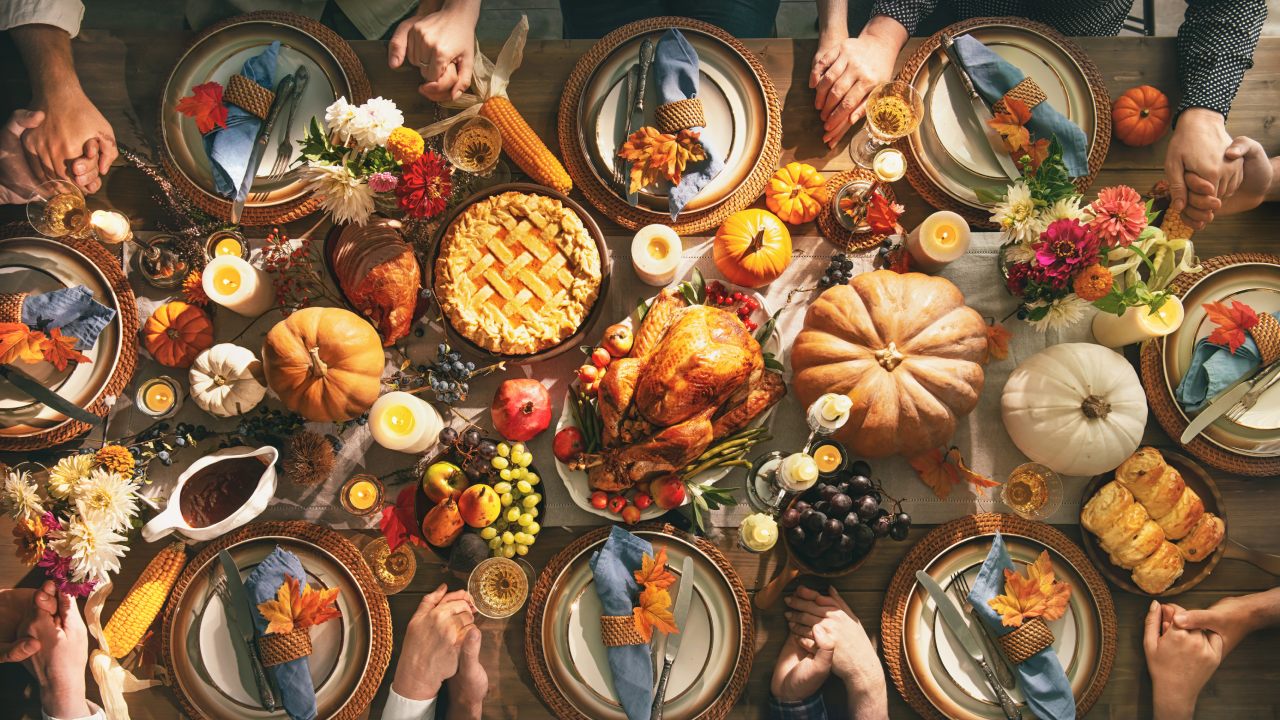This overhead Thanksgiving landscape photo captures a beautifully set table adorned with an array of traditional elements. At the center of the table sits a light and dark brown roast turkey on a white plate, surrounded by vegetables. Flanking the centerpiece are various pumpkins in shades of white, light orange, and darker orange, adding a fall festive touch. The table is laid out for eight people, with three place settings on each side and one at each end, all featuring white plates atop brown placemats, complemented by light blue napkins wrapped with brown rings and adorned with orange leaves.

In addition to the turkey, the spread includes a visible pie, a gravy boat, a fruit platter, a plate of bread rolls, and a round brown plate with loaves of bread. Decorative candles are lit, and colorful flower arrangements add to the festive ambiance. Hands can be seen extending into the frame, as if the assembled guests are holding hands in a moment of gratitude, reflecting the communal spirit of the occasion.